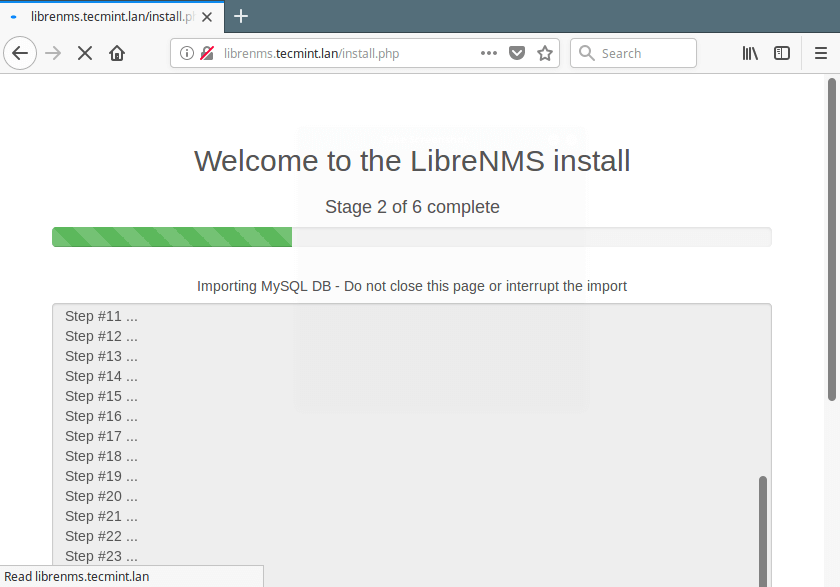A screenshot of a web page is displayed, revealing various browser elements and the content of a web-based application. At the top of the image, browser tabs are visible; one tab is active, while another tab to the right is blue with a plus sign for opening new tabs. Navigation controls including the back button, forward button, a close (X) button, and a home button are also present. The web page URL shown is "librems.techmed.lan.php," accompanied by a lock icon with a red strike-through, indicating a potential security concern. 

Below the address bar, a white search field and a bookmark tab are displayed. Dominating the center of the web page, a large header reads, "Welcome to the Libre NMS Install." The installation process is at stage 2 of 6, with a green progress bar filling approximately 30% of the status indicator. 

A grey scroll bar on the right side suggests additional content is available below the visible window. Immediately below the green progress bar, a message reads, "Importing MySQLDB. Do not close this page or interrupt the import." A list of steps is partially visible, starting from step number 11 and continuing to step number 23, detailing the installation procedure's current operations.